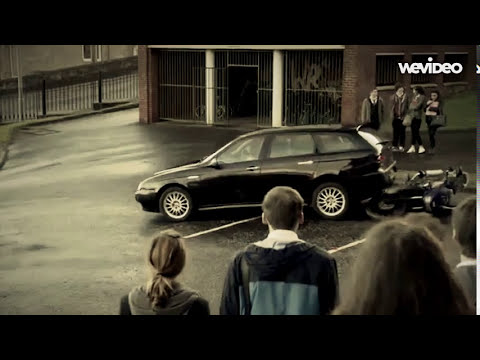The image showcases a black hatchback car in the center, positioned in a parking lot with diagonal white lines. The car appears mid-action, potentially having run over or backed into a blurry, tipped-over motorcycle lying on the shiny, wet ground. The scene is framed by black horizontal borders at the top and bottom, indicative of a video still. In the foreground, the backs of five people are visible, including a tall man in a navy and light blue jacket with a hood, a woman with a ponytail, and individuals with blondish hair. Across the parking lot, four other individuals, seemingly women dressed in black, are also observing the scene. The parking lot is situated near a building characterized by vertical bars, white pillars, and brown stonework, and a wrought iron fence is visible in the upper left corner of the image. The overall impression is that of an accident site, with onlookers gathered to examine the unexpected event.